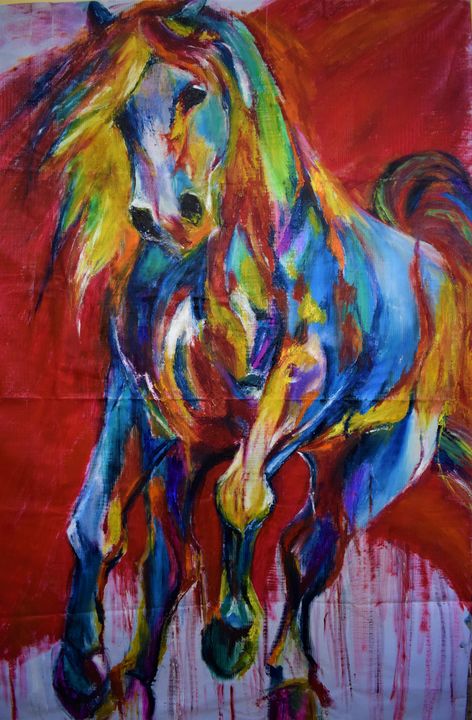The image depicts a vibrant painting of a horse galloping furiously forward, centered prominently with its hooves raised as if in mid-stride. The horse's body is an explosion of colors, including hues of blue, green, yellow, gold, orange, purple, red, pink, and white, giving it a rainbow-like appearance. Its mane and tail are depicted flowing as if caught in motion. The background of the painting transitions from white in the top left corner to a predominantly red center, with the red color seeming to bleed downward over lower sections of white. Blood-like streaks are visible dripping from the bottom of the horse, adding a dramatic and intense element to the artwork. The overall style creates a striking visual contrast, with the horse appearing almost as if it is running towards the viewer, vivid and full of dynamic energy against the dramatic backdrop.